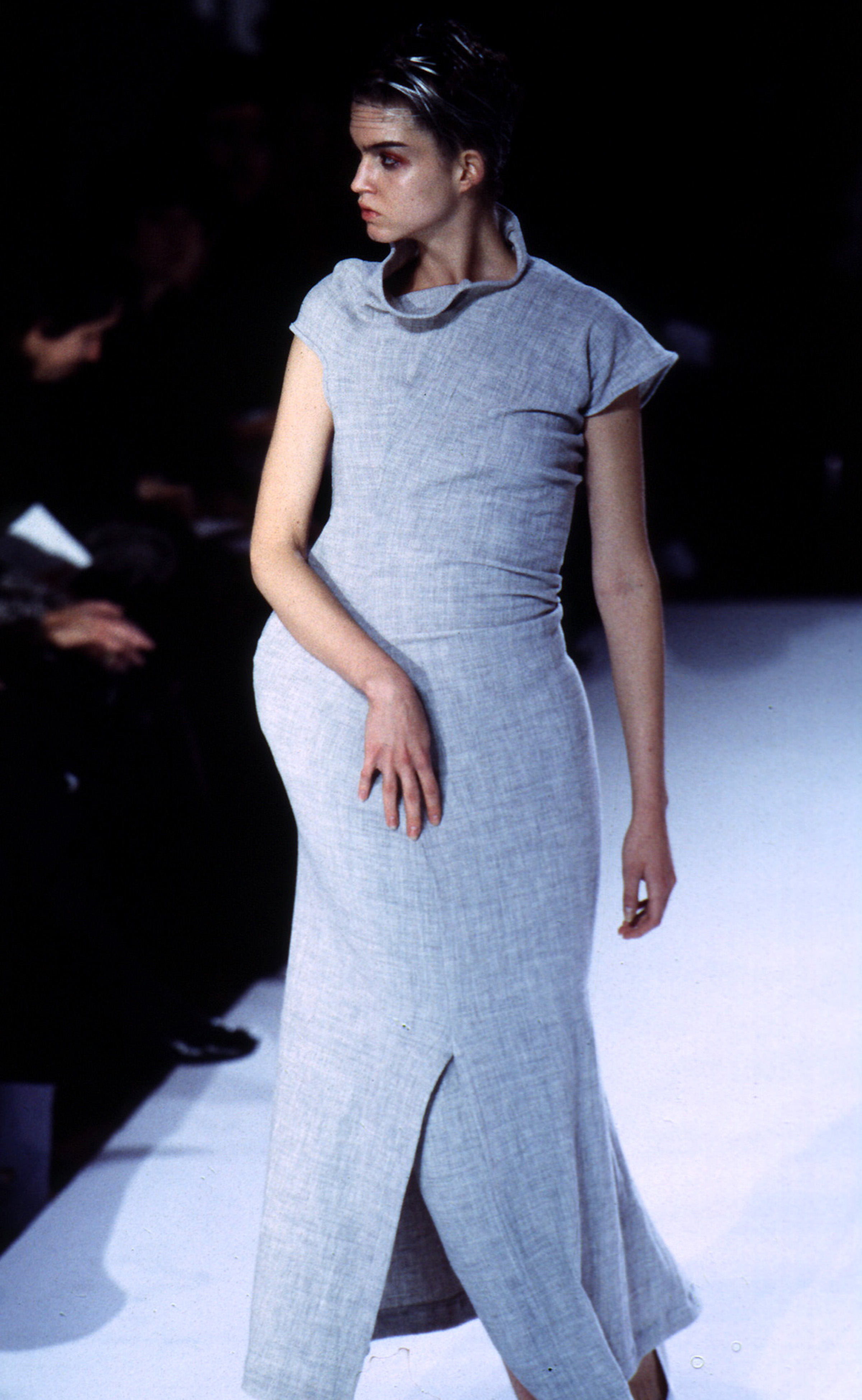The image depicts a pregnant model walking down a well-lit, white runway, illuminated against a dark background. She has black hair, which is either pulled back or styled with light highlights, and a light to tanned skin complexion. The model is adorned in a light blue, possibly denim-type dress with short or cap sleeves and a slit reaching up to her knees. Her makeup is subtle yet noticeable, featuring eyeliner. She strides confidently, looking to her right, while faint silhouettes of onlookers can be glimpsed along the sides of the runway. The overall scene, despite the dark backdrop, captures the bright and clear essence of the fashion show setting.